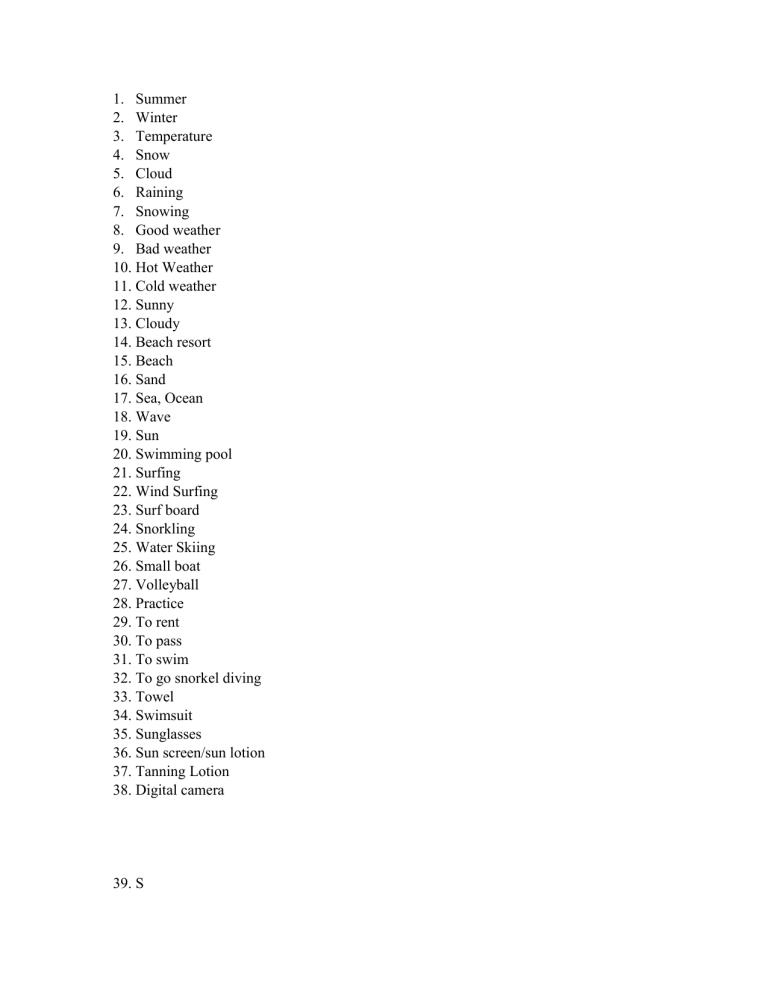This image captures a text file displayed on a white background, which could be a PDF or another type of document viewed on an unspecified device. The text is presented in black and is organized as a numbered list, extending to item 39. The list appears unfinished as the last entry is labeled "39. S," suggesting continuity. The list includes a variety of seasonal and vacation-related terms, potentially representing activities or items for a tropical getaway. The entries are:

1. Summer
2. Winter
3. Temperature
4. Snow
5. Cloud
6. Raining
7. Snowing
8. Good weather
9. Bad weather
10. Hot weather
11. Cold weather
12. Sunny
13. Cloudy
14. Beach resort
15. Beach
16. Sand
17. Sea, ocean
18. Wave
19. Sun (like the sun in the sky)
20. Swimming pool
21. Surfing
22. Windsurfing
23. Surfboard
24. Snorkeling
25. Water skiing
26. Small boat
27. Volleyball
28. Practice
29. To rent
30. To pass
31. To swim
32. To go snorkel diving
33. Towel
34. Swimsuit
35. Sunglasses
36. Sunscreen/Sun lotion
37. Tanning lotion
38. Digital camera

The entries suggest an emphasis on weather, seaside activities, and essential items for a beach vacation, providing a comprehensive overview of what one might consider for planning such a trip.